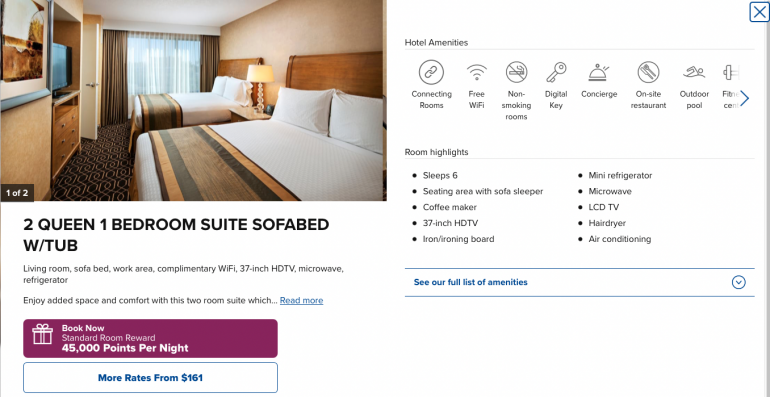This listing is for a suite featuring two close-set queen beds, separated by a polished wooden nightstand with a glossy finish. A desk lamp with an orangeish-yellow shade adorns the nightstand. The room's walls are predominantly white, transitioning to a tan-colored wallpaper on the left side. Directly in front of the beds, a TV is set into a wall recess, complemented by wooden drawers with silver handles. The oak-stained headboards exhibit a nuanced dark brown coloration with lighter brown streaks.

The back wall is similarly dark brown, matching the color theme of the headboards. The windows feature white curtains overlaid with dark gray drapes on both sides. The white bedspreads have a decorative end section featuring alternating bands of gold, black, tan, and brown.

Below the image, there's textual information describing the room: "One of two." Additional text reads, "Two queen one-bedroom suite sofa bed with tub." It includes details such as, "Living room with sofa bed, work area, complimentary Wi-Fi, 37-inch HDTV, microwave, and refrigerator." A prompt encourages potential guests to "Enjoy added space and comfort with this two-room suite," followed by an ellipsis and a link labeled "Read more."

A booking section includes a white gift icon with the text, "Book now standard room reward 25,000 points per night," positioned in a violet rectangle. Below that, another white rectangle with a blue border states, "More rates from $161," in blue text.

Amenities on the right side are listed with corresponding icons: "Connecting rooms" (chain link icon), "Free Wi-Fi" (Wi-Fi symbol), "Non-smoking rooms" (crossed-out cigarette), "Digital key" (key icon), "Concierge" (concierge bell), "On-site restaurant" (knife and fork), "Outdoor pool" (person treading water), and partial icon for another feature.

Room highlights are presented in bulleted format: sleeps six, mini refrigerator, seating area with sofa sleeper, microwave, LCD TV, coffee maker, 37-inch HDTV, hairdryer, iron/ironing board, and air conditioner.

At the bottom, dark blue bands enclose the text, "See our full list of amenities," with an arrow symbol indicating a dropdown. The top right features a blue square with an "X."